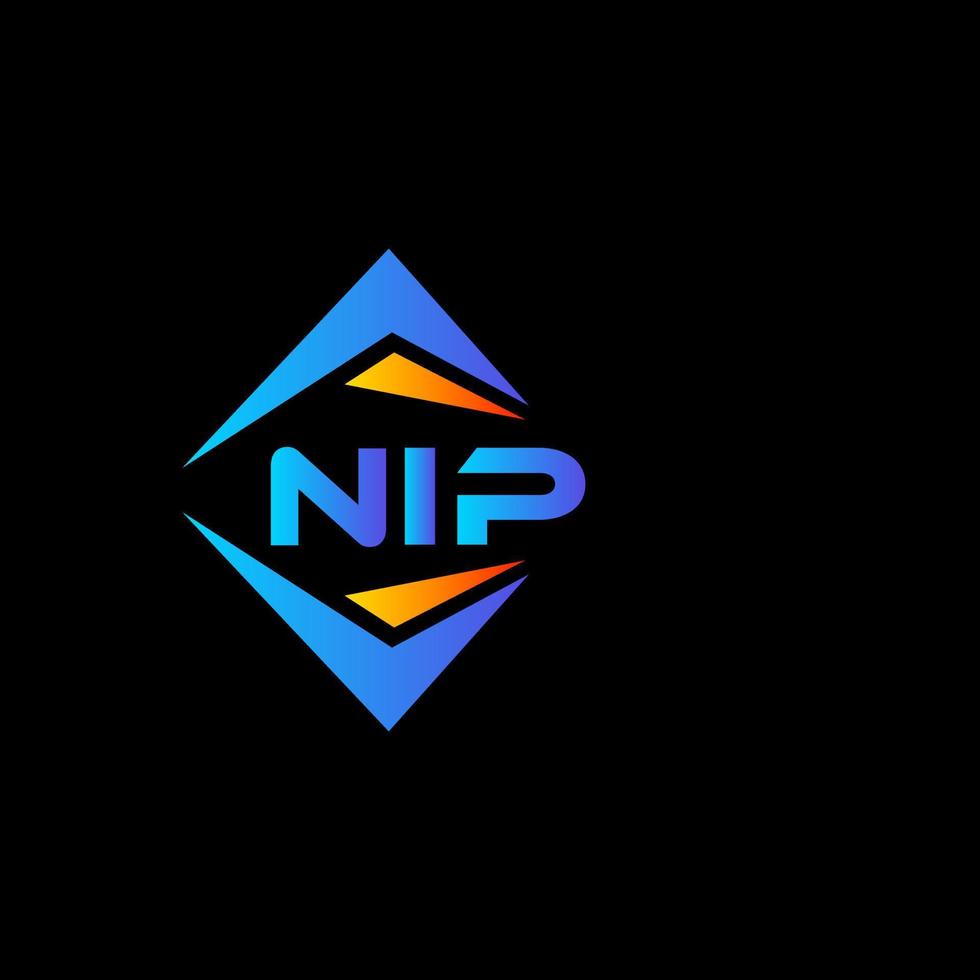The image features a minimalistic graphic design logo set against a solid black background. Positioned slightly to the left of the center, the logo is composed of geometric shapes and the letters "N-I-P." The diamond-shaped structure is formed by two large bright blue triangles with boomerang-like cutouts at the bottom, mirroring each other above and below a pair of smaller orange triangles that gradient from a bright to darker orange. The orange triangles point towards the right, with one above and one below the central letters. The bold letters "N-I-P" are in matching bright blue bubble letters, with a notable design in the letter 'P' where the top does not connect, resulting in an open loop.